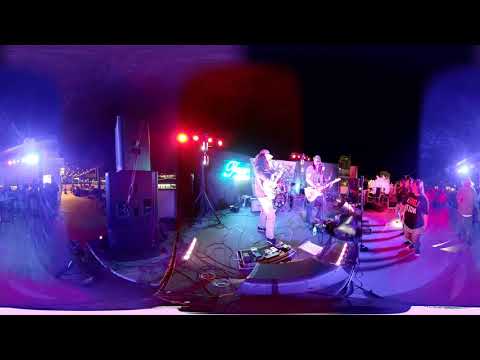The image captures an outdoor rock concert, evident from the dirt ground and night sky. Central to the scene is a stage with two male performers: one singing and the other rocking out on a guitar, both with long hair. The stage is adorned with vibrant neon lights in blue, red, and purple, illuminating the band and creating an electric atmosphere. Big speakers flank the stage, intensifying the music's impact. Behind the band, there's an illuminated but blurry sign, and spotlights shine from behind, casting dramatic glows. The left side of the image features a woman with an indistinct shirt graphic, near what appears to be a concession stand. The audience, mostly clad in jeans, crowds the right side, standing close in a pit area, clearly engrossed and rowdy. The image is fuzzy, with edges obscured by darkness and motion blur, highlighting the lively and chaotic essence of a nighttime concert experience.